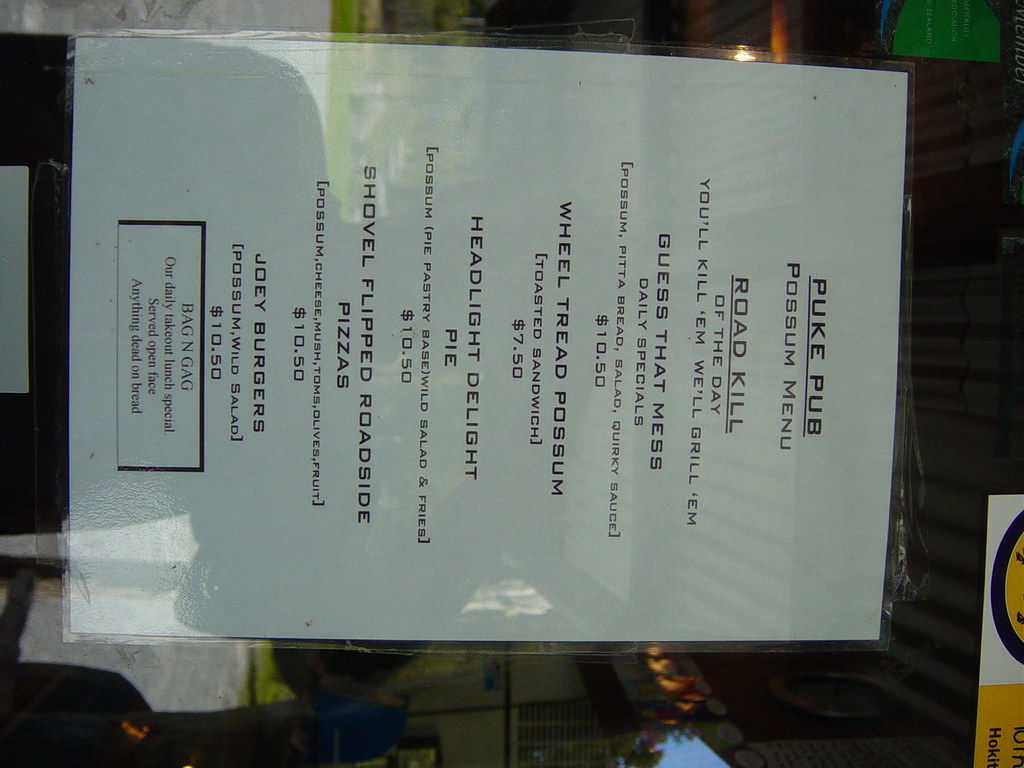The image captures a menu adhered sideways to a glass door or window using clear tape. The menu, printed on a white sheet of paper, features the bold, underlined title "Puke Pub." The quirky and unconventional items listed include "Post some Menu," "Roadkill of the Day" with the tagline "You'll kill him, we'll grill him," and "Guess That Mess" as daily specials priced at $10.50. Other offerings are "We'll Trade Possum" toasted sandwich for $7.50, "Headlight Delight Pie," and "Possum Pie Pastry" which comes with a pastry base, wild salad, and fries for $10.50. The menu intriguingly concludes with "Shovel Flipped Roadside Pizzas" and additional unspecified items.